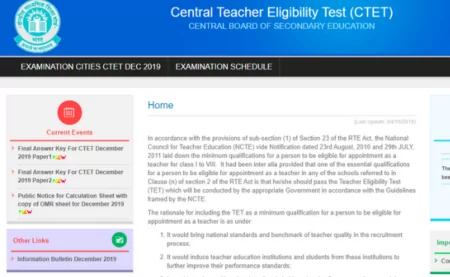This image is a screenshot from a website, showcasing a specific layout and design related to the Central Teacher Eligibility Test (CTET) and the Central Board of Secondary Education (CBSE). The top inch and a half of the image features a dark blue border, followed by an inch of black, and the remainder is predominantly white. Within the blue border, there is a barely legible, light blue stamp from a school. 

In the center of the image sits a white book. Overlaid on this book, starting in the center, is white text with large capital letters displaying "CENTRAL TEACHER ELIGIBILITY TEST" accompanied by the abbreviation "CTET." Below this, in smaller capital letters, is "CENTRAL BOARD OF SECONDARY EDUCATION."

On the left side of the black border, in all-capital white letters, it reads "EXAMINATION CITIES, CTET, DEC 2019." A small vertical gray line separates this from the next segment. Following the line, it continues with "EXAMINATION SCHEDULE," also in all-capital white letters, then another small vertical gray line.

Below, on the left side of the white background, there is a light blue rectangle extending about two inches, containing a red circle with a white calendar outline. Below this icon, in red text, it says "CURRENT EVENTS," with a red underline. Adjacent to this, three red arrows point to the right, accompanied by two lines of black text. Under this section, there is a small white space followed by another light blue rectangle that says "OTHER LINKS" in red text. To the right of this, a green circle with a white interior and a red underline appears, with the black text stating "INFORMATION BULLETIN DECEMBER 2019."

Further to the right, the background is entirely white. In the top corner, the word "HOME" is displayed, followed by a thin line. Below this are approximately ten lines of paragraph text, concluded by two additional lines, and markers labeled "1" with a line next to it, and "2" with two lines beside it.